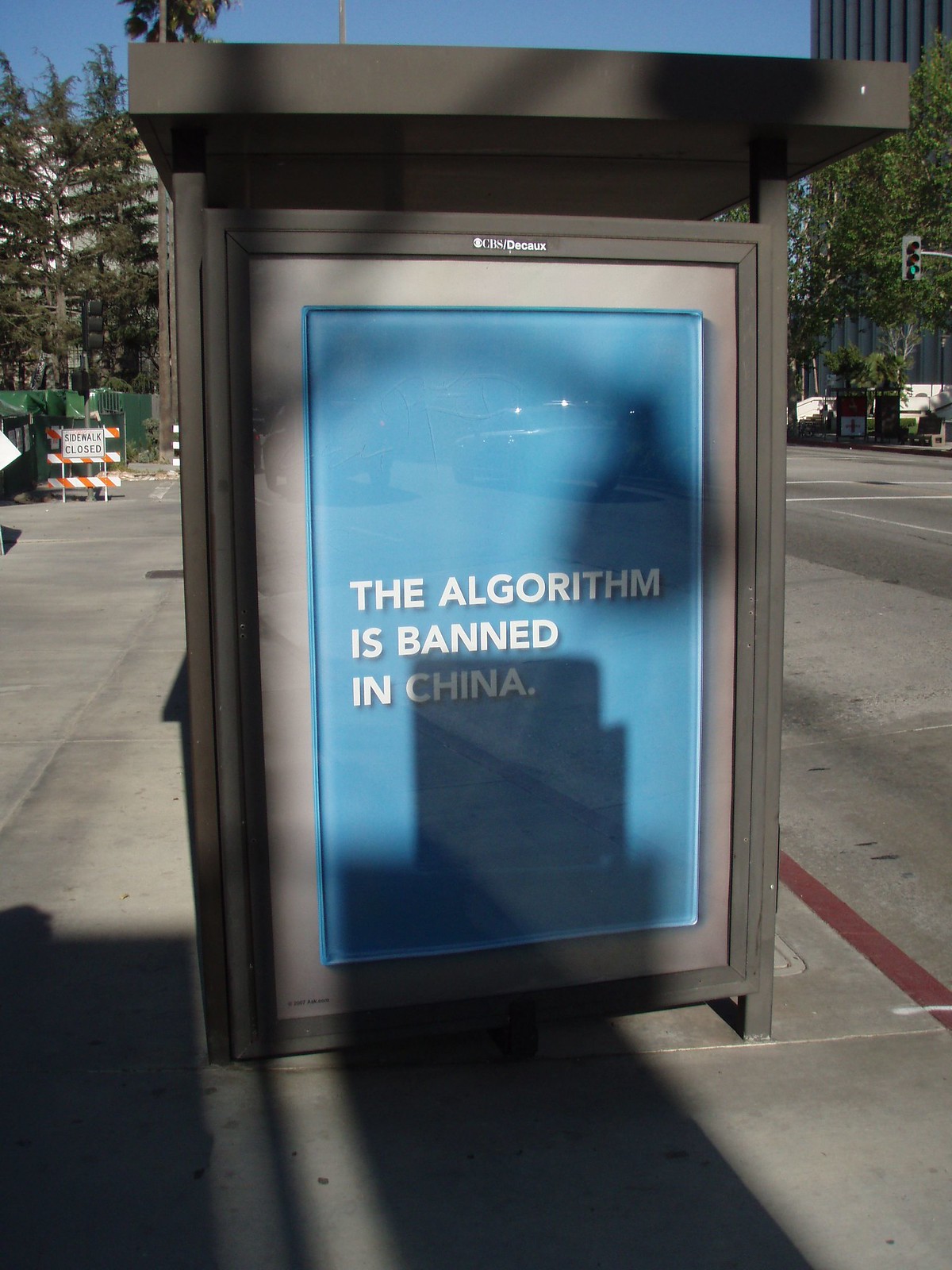This photograph appears to be taken with a handheld phone, depicting a bus stop situated in an urban area. The focal point is the side of the bus stop, which traditionally features advertisements or large posters encased behind thick glass or plexiglass. In this instance, a blue poster with white, sans-serif text boldly states, "The algorithm is banned in China." 

Above the poster, there is a small marker that reads "CBS/DECAUX," indicating either the management of the bus stop or the entity that owns the advertising rights to this particular display space. The environment surrounding the bus stop suggests a bustling city atmosphere, further emphasized by the contemporary design and maintenance of the advertisement structures.